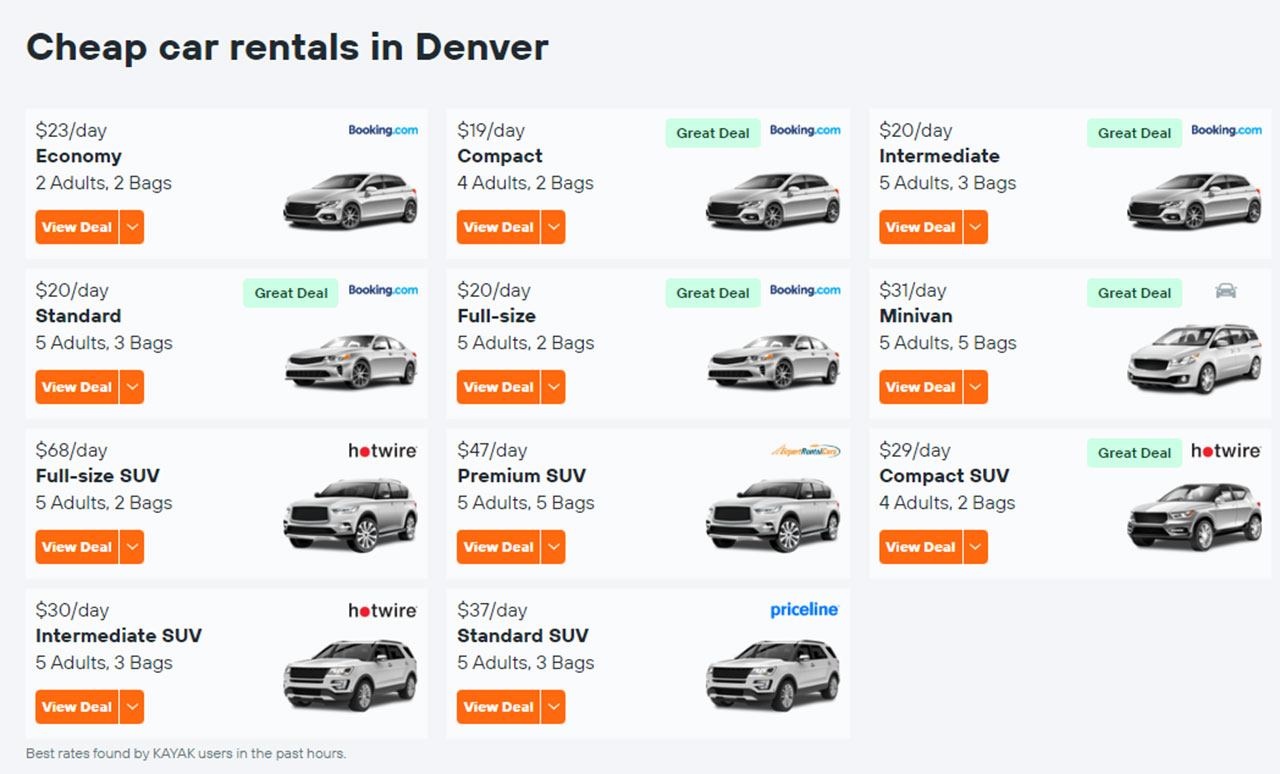This image is a detailed screenshot of a car rental comparison, set against a gray background. At the top left, in black print, the text reads "Cheap Car Rentals in Denver," with the "C" in "Cheap" and the "D" in "Denver" capitalized.

The screenshot is divided into three distinct panels, each displaying various car rental options in rectangular boxes. 

**First Panel:**
1. **Booking.com:** $23/day, Economy, 2 adults, 2 bags.
2. **Booking.com:** $20/day, Standard, 5 adults, 3 bags, labeled as a great deal.
3. **Hotwire:** $60/day, Full-Size SUV.
4. **Hotwire:** $30/day, Intermediate SUV.

**Second Panel:**
1. **Booking.com:** $19/day, Compact, labeled as a great deal.
2. **Booking.com:** $20/day, Full-Size, labeled as a great deal.
3. **Expert Rental Cars:** $47/day, Premium SUV.
4. **Priceline:** $37/day, Standard SUV.

**Third Panel:**
1. **Booking.com:** $20/day, Intermediate, labeled as a great deal.
2. **Hotwire:** $31/day, Minivan, labeled as a great deal.
3. **Hotwire:** $29/day, Compact SUV, labeled as a great deal.

The text details the pricing, vehicle categories, passenger and luggage capacities, and occasionally, the designation of "great deal" to highlight value offers, providing a comprehensive guide for potential car renters.